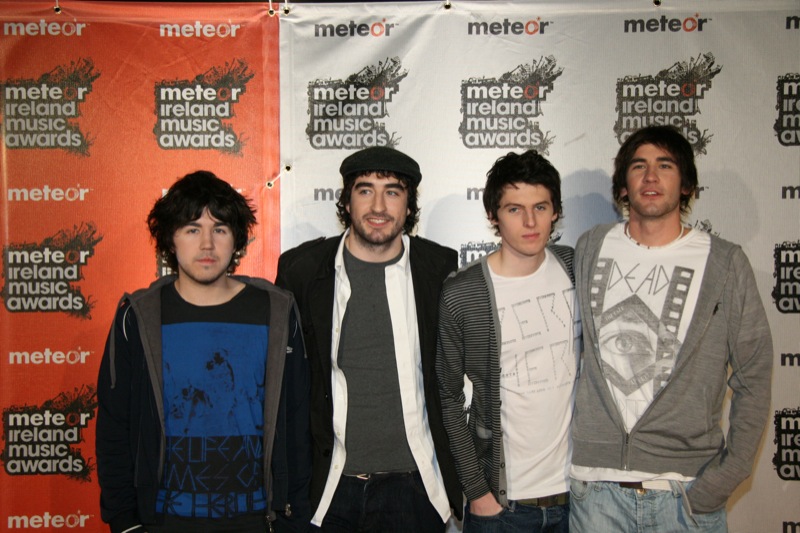In this image, four young Caucasian men, likely in their early twenties, stand closely together, smiling in front of a backdrop for the Meteor Ireland Music Awards. The backdrop features repetitive text with "Meteor Ireland Music Awards," with the left side in a red or orange color and the right side in white. From left to right, the first man is the shortest, has longish hair, dark eyebrows, dark eyes, and stubble, and is dressed in a blue and black shirt with a hoodie. The second man is wearing a cap over his long, curly hair, a coat over a white shirt layered with a t-shirt, and dark trousers; he has heavy eyebrows, a close-cropped beard, and is smiling. The third man has shorter dark hair, possibly blue eyes, and is dressed in a striped sweater over a white shirt with blue jeans. The fourth man, on the far right, has longish hair, dark eyebrows, dark eyes, a close-cropped beard, and is wearing a t-shirt that says "dead" with an eyeball graphic, a gray hoodie, and blue jeans. They appear to be musicians enjoying a proud moment, possibly after receiving an award, and their casual attire, including t-shirts, jeans, and sweatshirts, reflects their relaxed camaraderie.